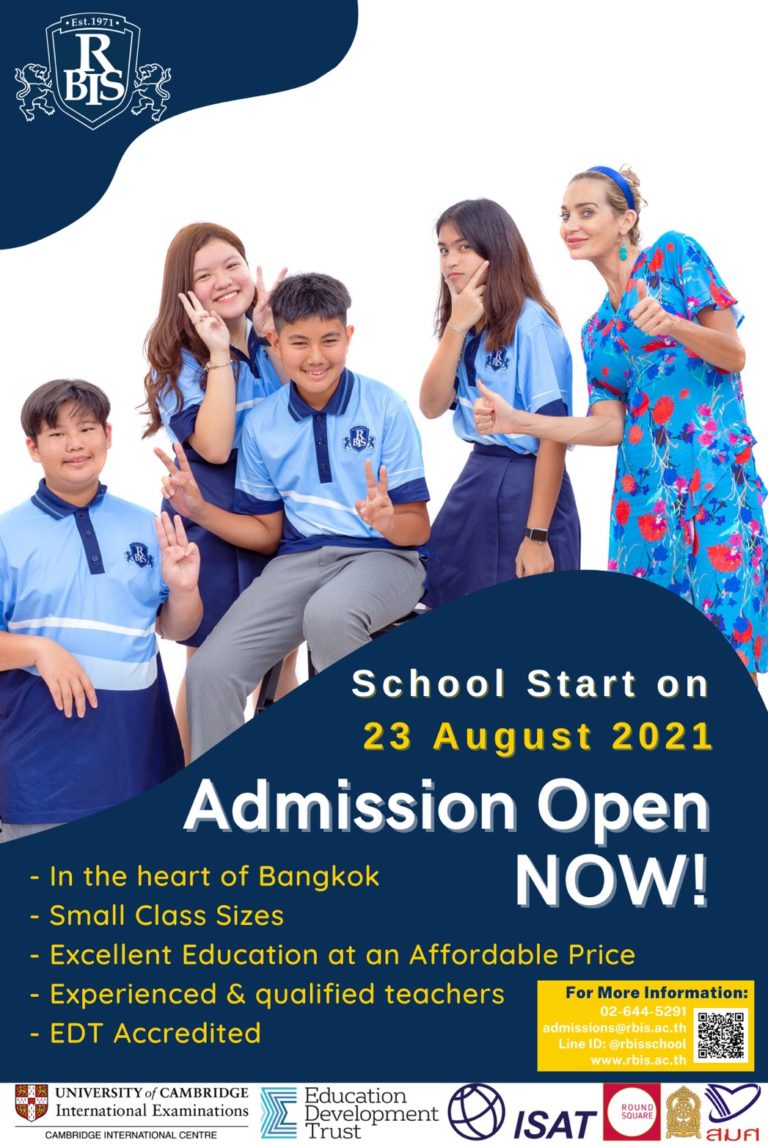In the image, the top left corner features a prominently raised logo that reads "East 1971 RBIS" against a dark blue background. Centered on the main page are photos of four students alongside their teacher. The female teacher, positioned on the right side, is enthusiastically giving a thumbs-up and is dressed in a vibrant blue dress adorned with red, pink, and dark blue floral patterns. The students, all in school uniforms, consist of three females and one male. The female students wear blue and white or light blue t-shirts paired with dark blue skirts, while the male student dons grey trousers. The background behind them is white, emphasizing the group.

At the bottom of the image, a dark blue section contains crucial information. On the right side, white text announces "School starts on 23 August 2021," with the date highlighted in yellow. Additionally, it states "Admission open now." 

The bottom left of the image features a yellow text block detailing the school's location "in the heart of Bangkok," and promotes "small class sizes," "excellent education at an affordable price," and "experienced and qualified teachers," noting the school's ADT accreditation. 

On the bottom right, the contact information is clearly displayed: phone number "02-644-5291," email "admission@srpis.ac.th," Line ID "srpis code," and the website "www.rpis.ac.th," alongside a black-and-white QR code for quick access. 

Lastly, logos and text for prestigious affiliations like "University of Cambridge International Examination," "Cambridge International Centre," "Educational Development Trust," "ISAT," and "Round Square" are displayed on the bottom left, underscoring the institution's credibility.